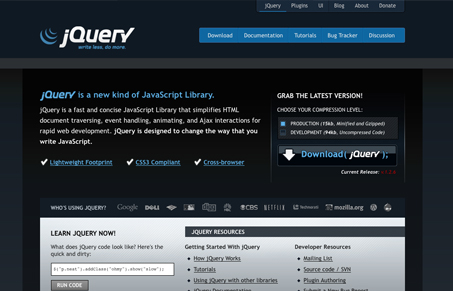**Image Description:**

The image appears to be a low-resolution screenshot of a web page, likely the homepage of a website related to jQuery given the textual elements present. The overall color scheme consists of a black background with primarily white and blue text.

At the very top of the page, there is a logo consisting of three blue curved lines pointing downwards, resembling a Wi-Fi signal icon typically found on the top bar of a smartphone. Next to this icon are the characters "jQuery" in a stylized format, where the initial 'j' is lowercase, followed by the capital letters "QUERY". This indicates that the website's focus is on jQuery, a popular JavaScript library.

In the upper right corner, there are several links, possibly leading to various sections or topics on the website. Although the text is unreadable due to poor resolution, one of these links is underlined in blue, which likely represents the currently active section.

Below the top bar, there is a row of blue buttons with white text. The first button might say "Dashboard", while another might say "Bug Tracker", although the exact text on each button is not entirely clear.

Further down, there is a text box with the heading "jQuery is a new kind of JavaScript library". Accompanying this text is a blue download button labeled "Download jQuery", which features a white downward-pointing arrow. Adjacent to this section, there are three bullet points accompanied by check marks. The visible text denotes that jQuery is lightweight and CSS compliant; however, the third point is unreadable.

Below that, another row of links is visible, though the specifics are indiscernible. 

Toward the bottom of the screenshot, there is a light gray box with the text "Learn jQuery Now". Beneath this box, there is a white input field that could be a search box or an email subscription field, paired with a gray button below it. Additional links are present, one possibly leading to a mailing list or tutorials, although their exact text is unclear.

Overall, the screenshot captures various key elements of the web page, indicating its purpose as a resource for learning and downloading jQuery.